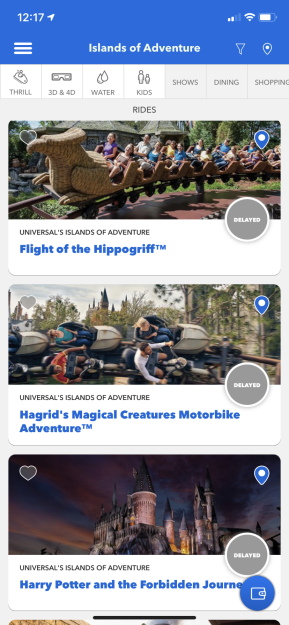In the image, we observe a mobile application interface displaying information about the Universal Studios’ Islands of Adventure theme park. The app is shown on a smartphone, indicated by the phone status bar at the top, showcasing the time, Wi-Fi signal, and battery percentage, along with a blue header.

Prominently, the header reads "Islands of Adventure" in white text, confirming the park's identity. Just below the header, there are clickable tabs that likely categorize different attractions and services in the park, labeled as Thrill, 3D and 4D, Water, Kids, Shows, Dining, and Shopping.

Below these tabs, the section titled "Rides" lists various attractions along with their current status. Featured rides include:
- **Flight of the Hippogriff**, shown with an image of a roller coaster and marked as "Delayed."
- **Hagrid's Magical Creatures Motorbike Adventure**, also marked as "Delayed."
- **Harry Potter and the Forbidden Journey**, similarly marked as "Delayed."

Each entry appears to offer a status update, possibly related to ride availability or wait times. The app interface is organized and user-friendly, designed to help visitors navigate the park and plan their activities effectively.